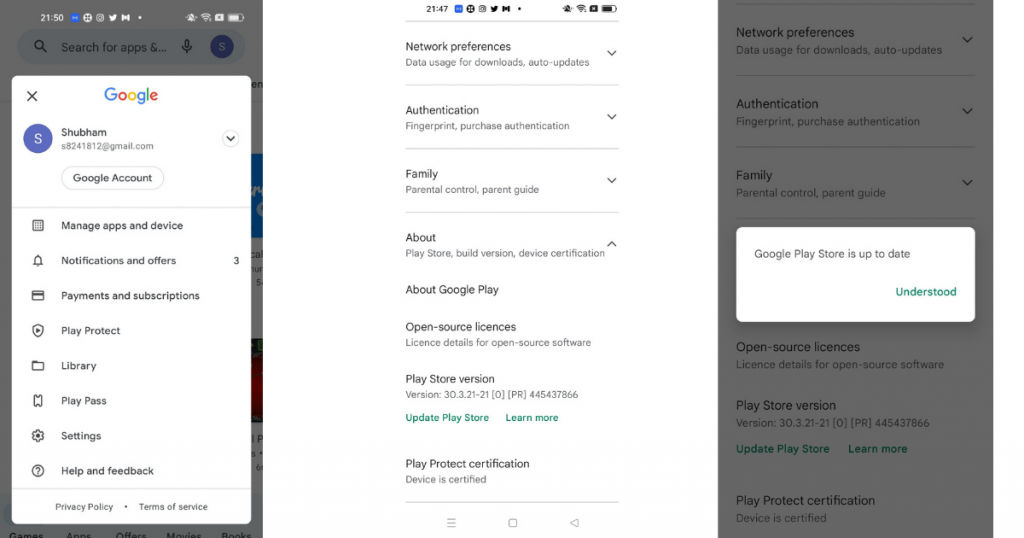This image shows a series of three phone screenshots displaying various settings and information screens within the Google Play Store app.

**Leftmost Screenshot:** 
- The time displayed is 21:50.
- At the top, there is a search bar with the placeholder text "Search for apps."
- The main section of this screenshot features a white background.
- Centered at the top, the word "Google" is shown.
- Below this, the name "Shubham" is displayed, along with their email address.
- The text "Google account" appears underneath the email.
- A line separates this section from several clickable options listed below:
  - Manage apps and device
  - Notifications and offers
  - Payments and subscriptions
  - Play Protect
  - Library
  - Play Pass
  - Settings
  - Help and feedback
- At the very bottom, there are links to the "Privacy policy" and "Terms of service."

**Middle Screenshot:**
- The time displayed is 21:47.
- This screen lists various setting categories from top to bottom:
  - Network preferences
  - Data usage for downloads
  - Auto updates
  - Authentication
  - Fingerprint purchase authentication
  - Family (which includes parental controls and parent guide)
  - About (currently expanded)
  - Play Store build version
  - Device certification
- The expanded "About" section provides details on:
  - About Google Play
  - Open source licenses
  - Play Store version
  - Play Protect certification

**Rightmost Screenshot:**
- The screen shows a notification stating that the Google Play Store is up to date.
- A green "Understood" button is present for acknowledging the information.